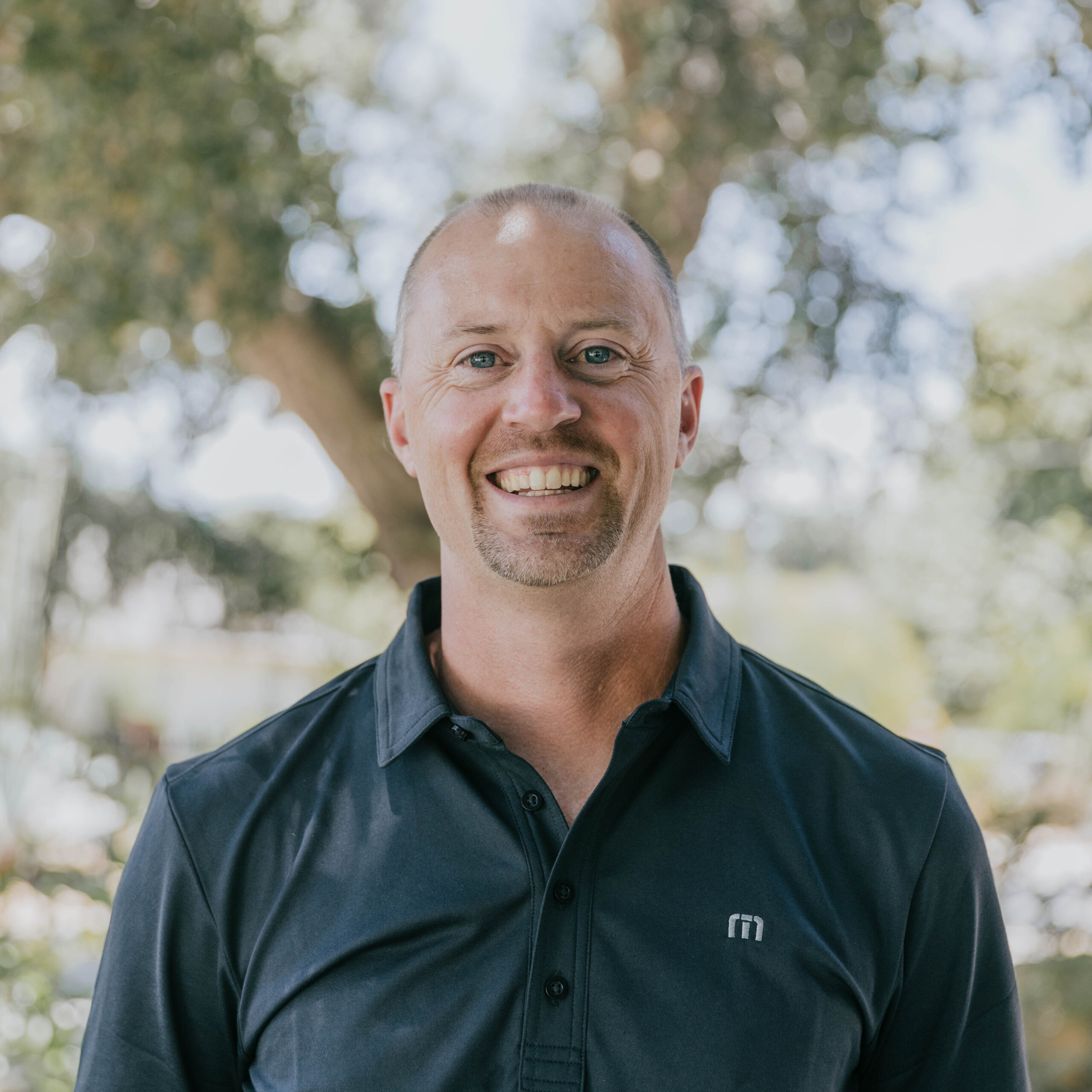The photograph, taken outdoors, prominently features a headshot of a Caucasian man in his forties, extending up to his chest. He has very short, slightly graying hair, particularly noticeable on the sides, and a bit of facial hair, with stubble around the goatee area. The man has bright blue eyes and is smiling widely, showing his teeth. He is wearing a very dark gray, almost black t-shirt with a distinctive "M" logo on it. The shirt has a collar and four buttons visible from the chest to the neck. In the background, which is blurry, there are trees and leaves, adding a natural element to the setting.